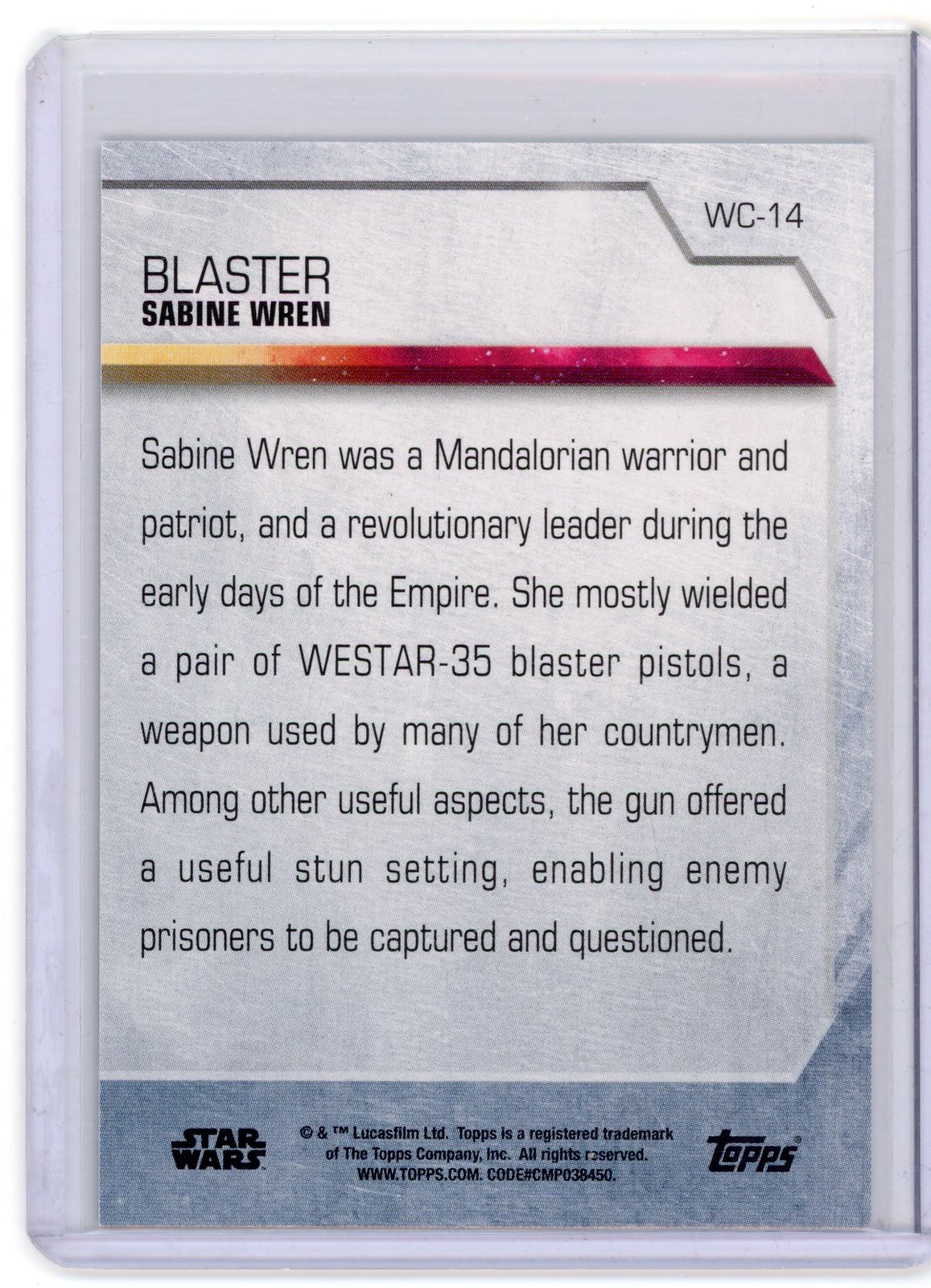This image is a color photograph of a collector card likely from TOPS, set against a gray, granite-like background. The card is in portrait orientation and features a blend of text and color graphics. At the top left, it prominently displays the word "BLASTER" in all caps, followed by "SABINE WREN" beneath it. A horizontal band with gold on the left and red on the right separates these headings from a detailed paragraph below. This paragraph describes Sabine Wren, a Mandalorian warrior, patriot, and revolutionary leader during the early days of the Empire. It highlights that she predominantly wielded a pair of Westar-35 blaster pistols, known for their useful stun setting, which allowed for the capture and interrogation of enemy prisoners. In the top right corner, set against the gray granite background, the card is labeled as WC-14 in black text. The bottom section features a blue denim-like background with the Star Wars logo in black on the left, intricate trademark and copyright information, and the TOPS logo on the bottom right. The card combines elements of graphic design and typography to create an informative and collectible piece.